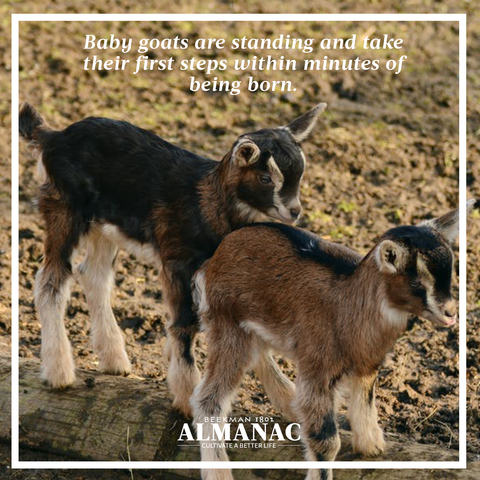The square photograph features two baby goats standing outdoors, framed by a thin white border. On the top of the image, white text reads, "Baby goats are standing and take their first steps within minutes of being born." At the bottom center, more white text says, "Beekman 1801 Almanac, Cultivate a Better Life." 

One baby goat, positioned in the front and slightly to the right, has a light brown coat with a distinctive black stripe running from its nose along its back. It also has a white underbelly and white legs. The second baby goat, standing behind the first and slightly to the left, has a darker black body with white legs and various tan spots. Both goats are looking towards the bottom right corner of the photograph, captured in a side profile that shows the detailed color variations and markings on their coats. The image combines realism with graphic design elements, portraying the innocence and curiosity of the young animals.